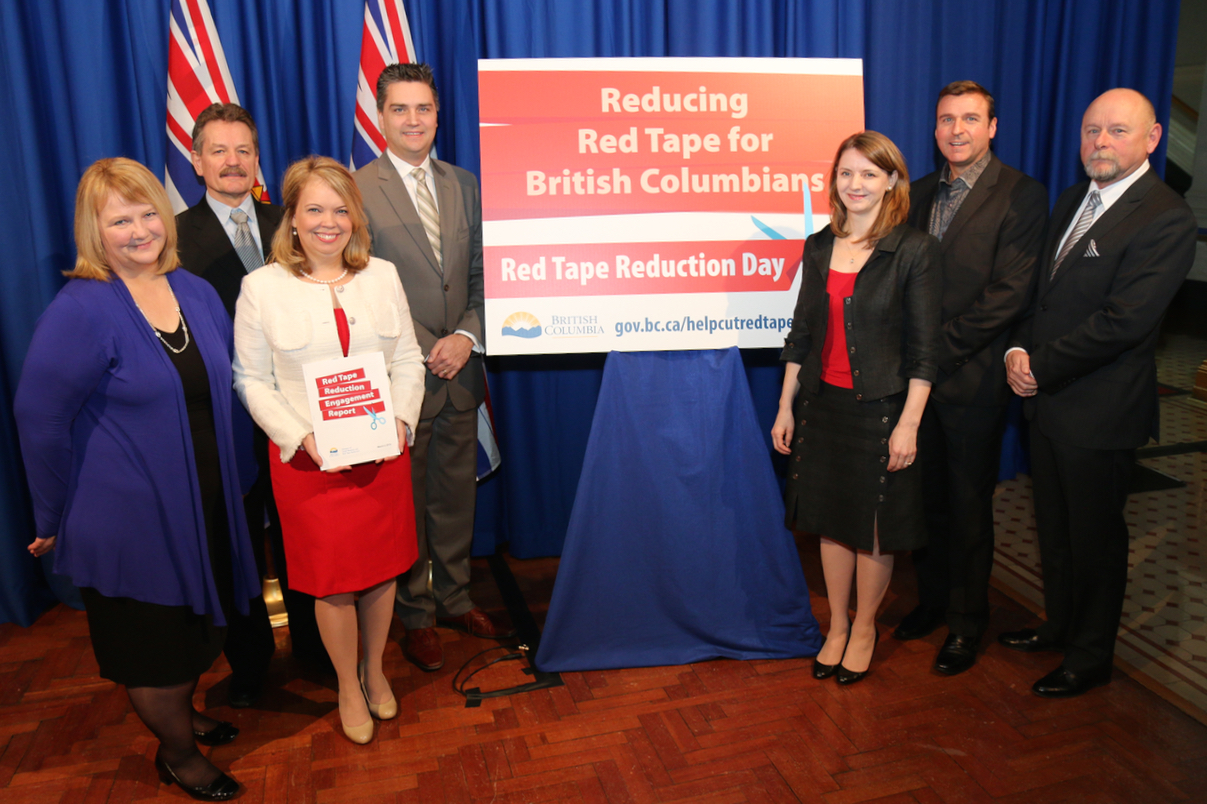In this detailed image, we see a group of seven individuals—three women and four men—dressed smartly and standing on a wooden floor. They are gathered around a prominent sign that reads, "Reducing Red Tape for British Columbians," with "Red Tape Reduction Day" written beneath it. This sign is centrally positioned in the photo. Behind the group is a blue curtain, flanked by two flags. The image is horizontal and rectangular in shape. Everyone is facing the camera and smiling, suggesting a formal yet celebratory occasion, likely taking place at a government meeting or event, in the middle of the day. The color palette includes brown, tan, black, gray, red, blue, white, and yellow. Additionally, a logo on the bottom left corner of the sign says "British Columbia" along with a web address, further emphasizing the official nature of the event.